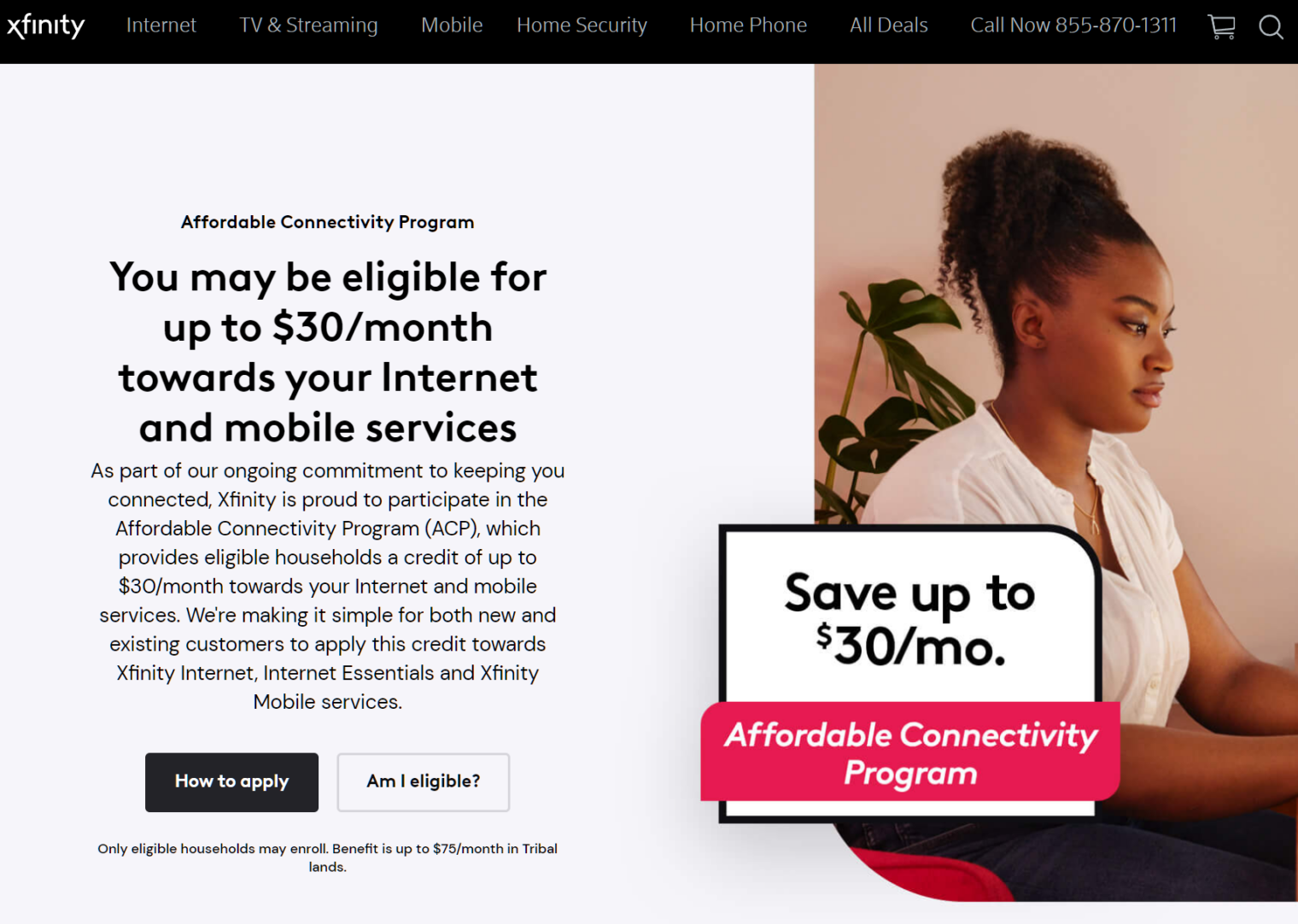This image is a detailed screenshot from a website advertising an "Affordable Connectivity Program." At the top, a black banner features various clickable items. The word "Xfinity" appears in bold white font in the top left corner, with a shopping cart icon and a magnifying glass icon towards the right end of the banner.

Central to the advertisement is a predominantly white background. On the right side, there is a photograph of a black woman with her hair pulled up, seated in a red chair. She is dressed in a white blouse and black trousers, with a cheese plant placed behind her. An information banner overlaps the photo, stating, "Save up to $30/mo." in bold text. Below this, a red banner reads "Affordable Connectivity Program" in white font.

To the left of the image, text on a white background provides more detail, beginning with "Affordable Connectivity Program: You may be eligible for up to $30/month towards your internet and mobile services." Additional information follows in smaller print.

At the bottom of this text, two buttons are displayed: a black button with white text labeled "How to Apply" and a white button with black text labeled "Am I Eligible?"